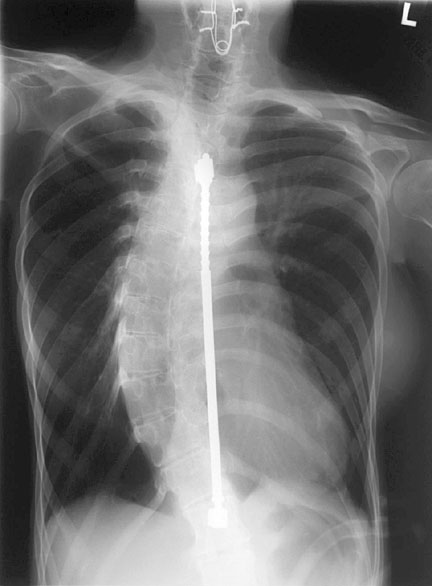This image is a detailed x-ray of a human torso, showing the chest and stomach areas, and capturing parts of the shoulders and neck. The x-ray prominently displays the ribcage and spine, with the bones appearing in shades of gray against a black background. Notably, the spine is slightly curved toward the left side and has a vertically oriented rod, which stands out as it is completely white, likely used for spinal correction. The image also includes foggy, silvery markings within the chest area, giving it a hazy appearance. Additionally, a bold, slightly tilted white letter "L" is visible in the top right corner of the image, marking the orientation.